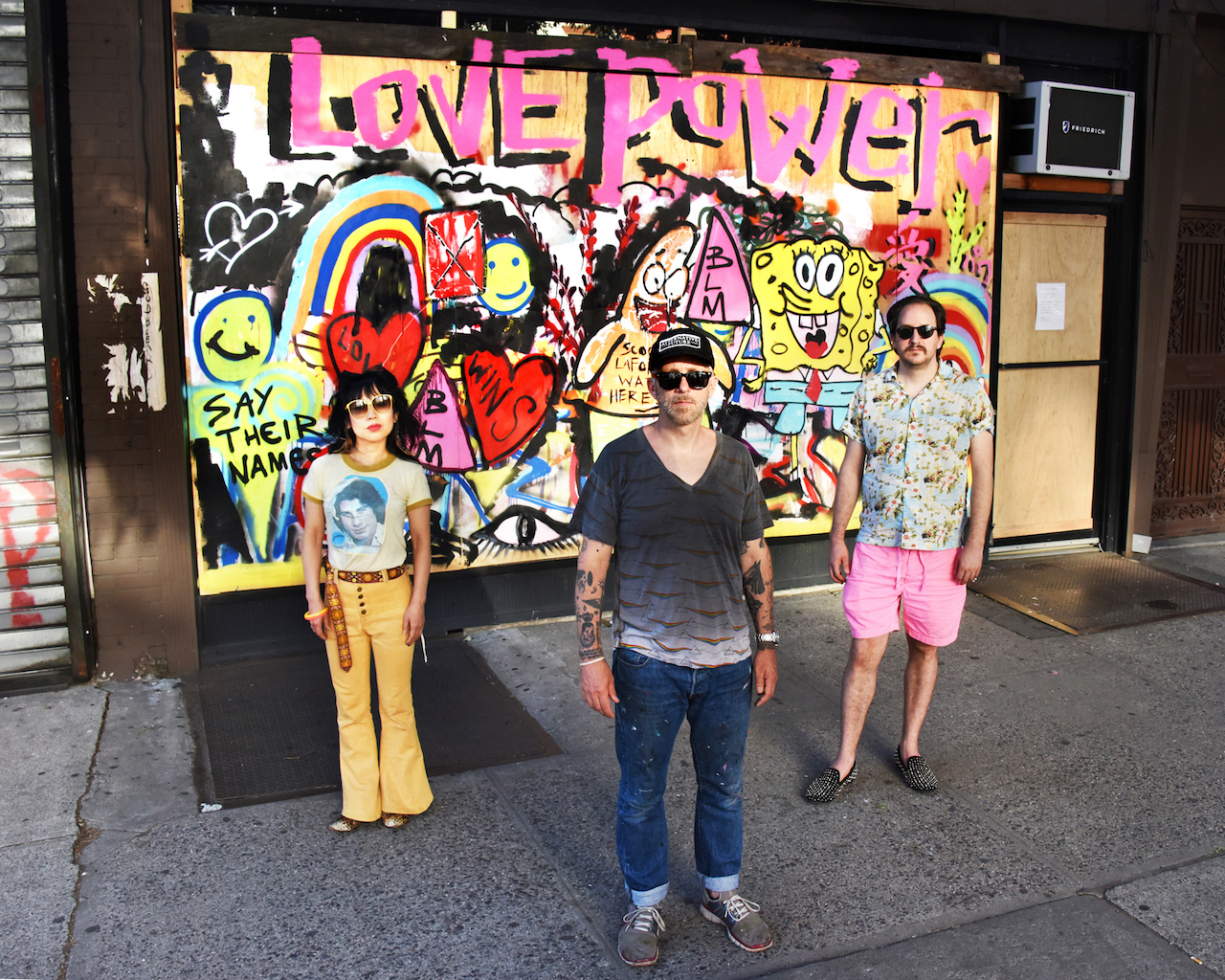The image captures three individuals, two men and a woman, standing on a sidewalk in front of a vibrant, graffiti-style mural painted on a boarded-up storefront. The mural prominently features the phrases "Love Power" in pink, "Love Wins," and "Say Their Names," along with numerous symbols and characters like SpongeBob SquarePants, Patrick, rainbows, smiley faces, and triangles with "BLM" (Black Lives Matter) written inside. The characters and motifs create a chaotic yet energetic art piece that exudes positivity and activism.

The people are casually spaced in a rough triangle formation, all wearing sunglasses. The woman, slightly shorter, sports a retro 1970s outfit: yellow bell-bottom pants, a light yellow t-shirt with a darker yellow trim on the collar and sleeves, and a geometric-patterned belt with orange and yellow circles. Her t-shirt features the face of, presumably, John Travolta. The man in the center wears a hat, heavily tattooed arms, jeans, and a plain dark t-shirt. The man on the right dons a floral print button-up shirt, pink shorts, and loafers or moccasins. Their eclectic appearances and relaxed stances suggest a fun and spirited atmosphere in alignment with the mural's themes.